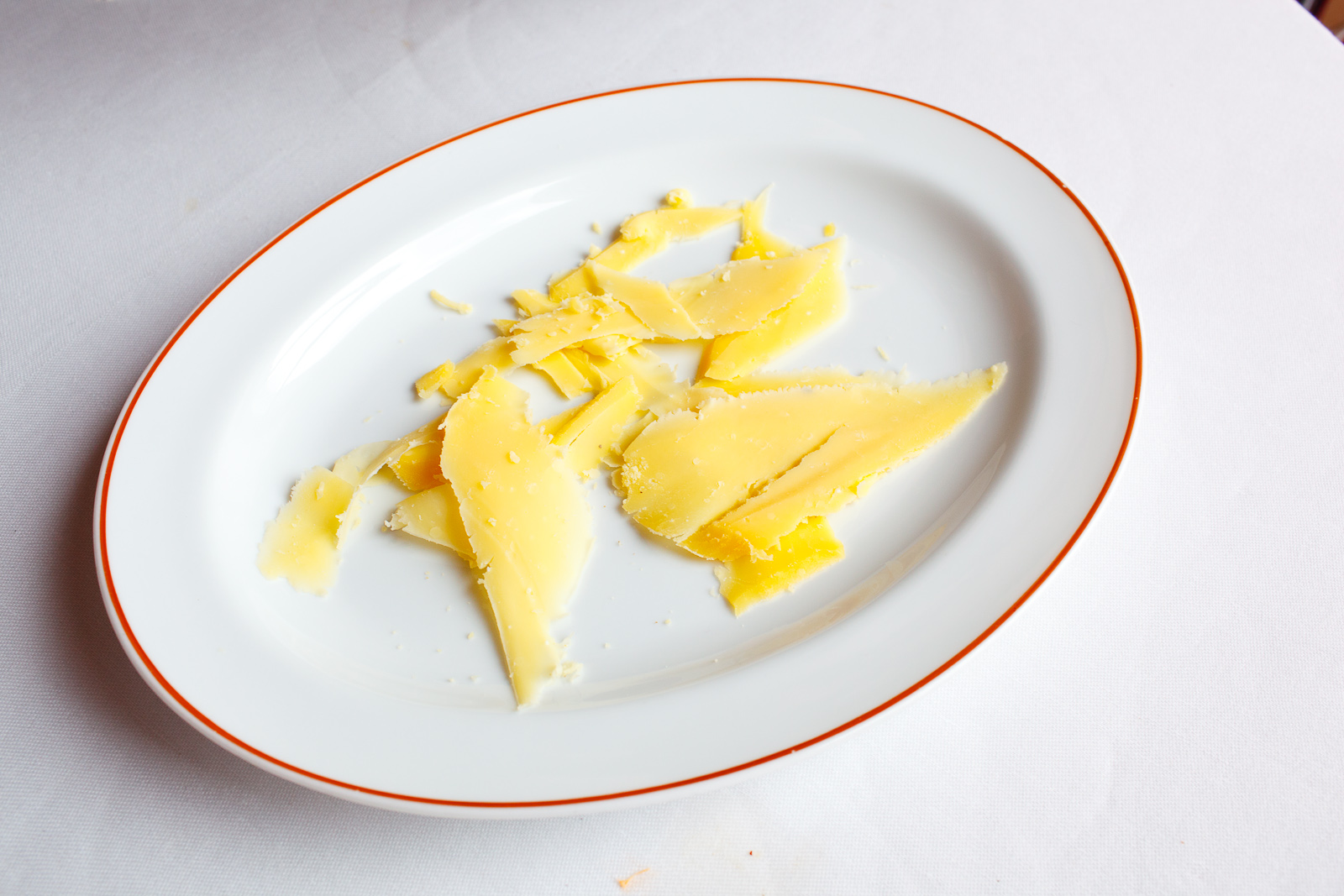The image depicts an oval ceramic plate with a smooth surface, featuring a thin, red border along its edge. The plate sits on a table adorned with a white tablecloth, which has visible creases and a small stain near the bottom center of the image. Reflecting a bit of light, the plate contains irregular shreds and flakes of yellow cheese, possibly Parmesan, scattered across its surface. In the upper right corner of the image, part of a brown chair is visible. There are a few crumbs on the plate, indicative of the nature of the cheese.